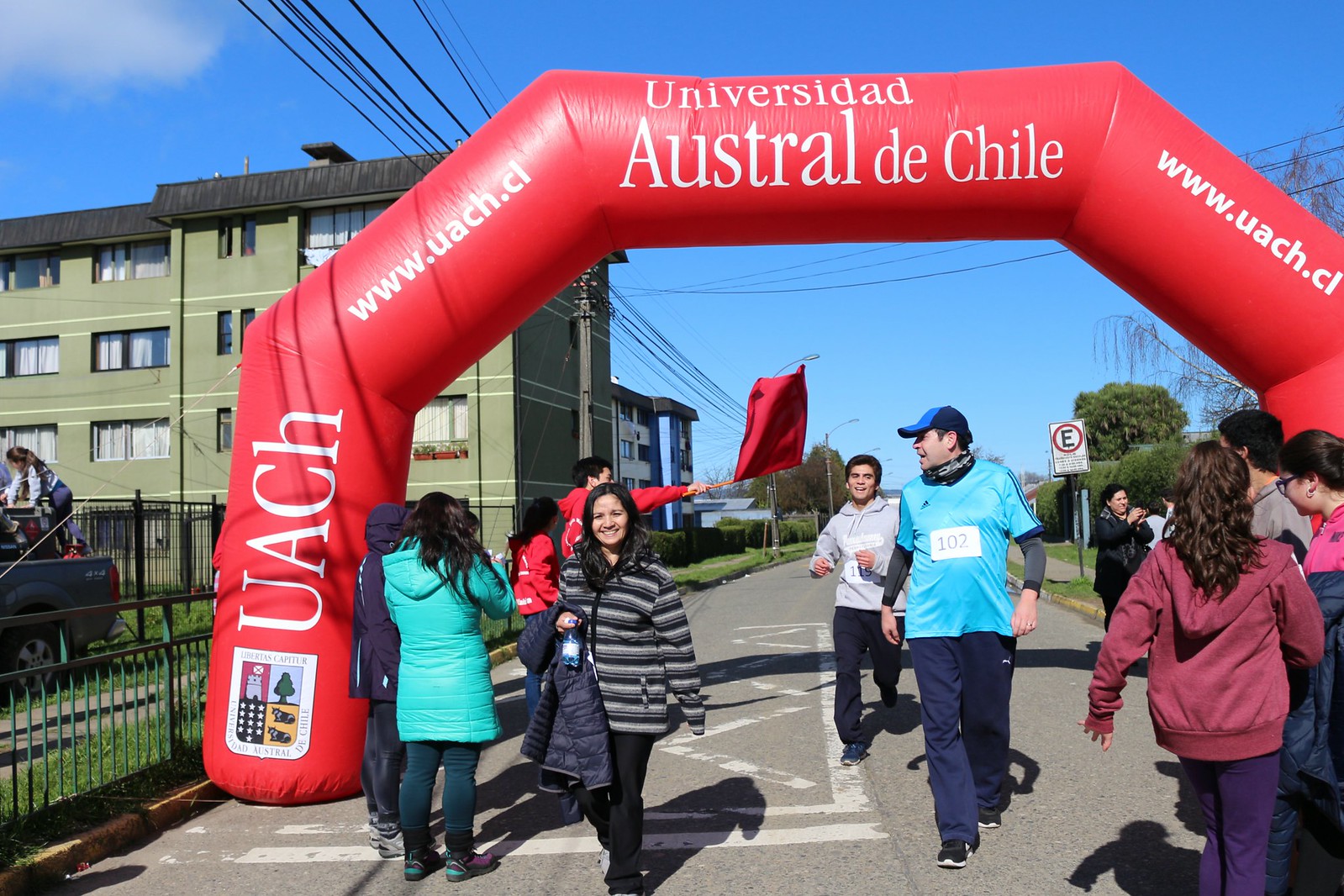The image depicts a vibrant scene at the finish line of a race event, set under a large, red inflatable archway that reads "Universidad Austral de Chile" with the website "www.uach.cl" prominently displayed. The finish line is crowded with participants and onlookers; a man in a red shirt holds up a red flag as a runner in a light blue shirt and a green, light blue, and black cap crosses the line. Close behind is another runner dressed in a gray hoodie. Among the crowd, some individuals are taking pictures, capturing the moment. The road, framed by green trees and a clear blue sky with a few white clouds, runs beneath an overpass marked with the university's banner. In the background, on the left, a brown building with a black roof stands behind a fence, along with a vehicle parked in what seems to be a lot. Additional details include visible electrical wires and a green building, adding to the everyday urban setting illuminated by daylight, enhancing the color and clarity of the scene.